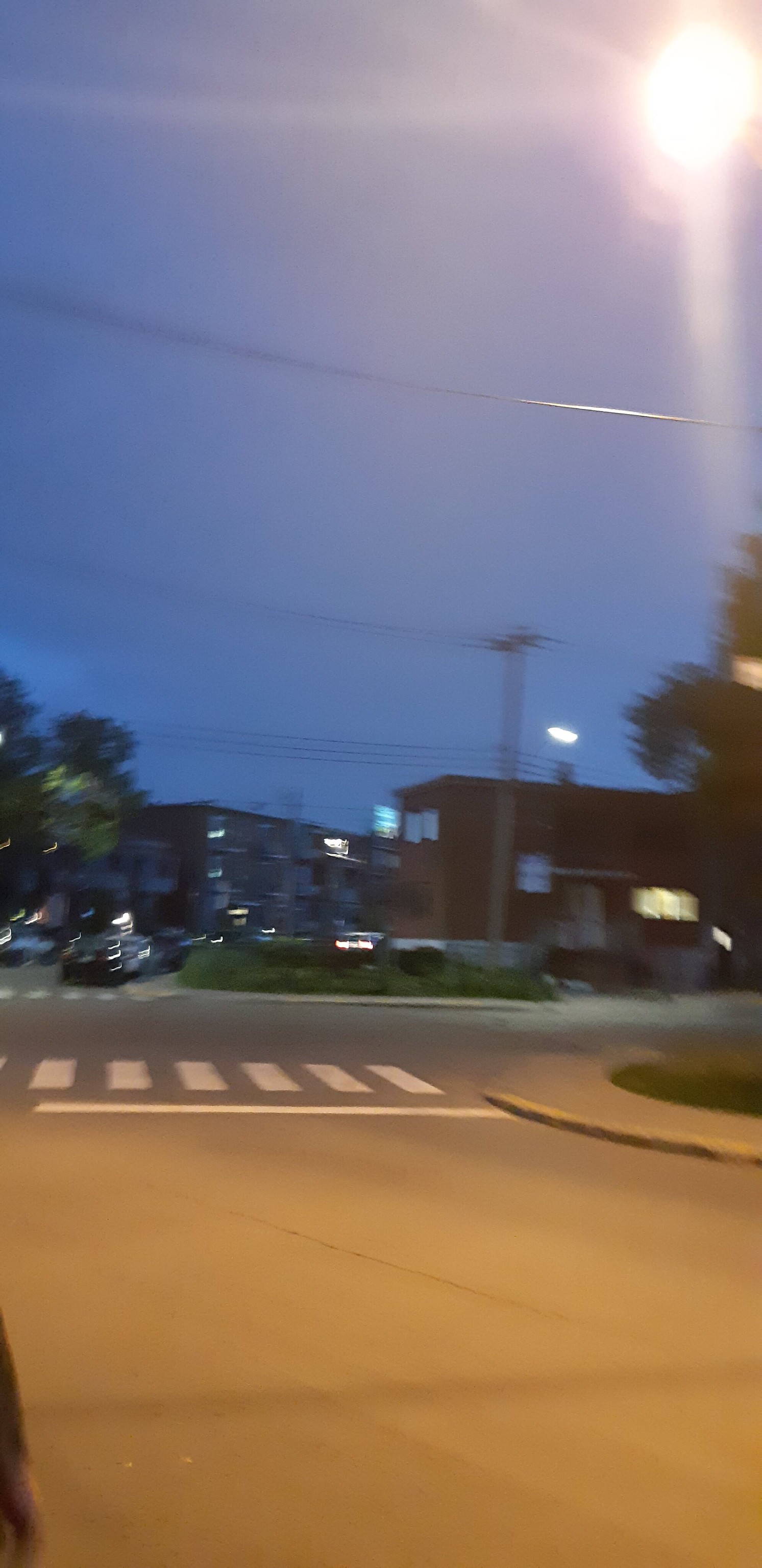The image is a large, vertically-oriented rectangular photo of a street at night, taken from inside a moving car. The street features a white line with six vertical rectangular boxes above it, possibly indicating crosswalks. The road appears to allow for straight, left, or right turns, with no stop signs or traffic lights visible—it's a "watch out" kind of area. On the right side, a big concrete curb frames some grass. The sky is adorned with a bright moon in the top right corner, next to a streetlight. In the distance, several rectangular buildings, possibly apartments, are seen. Although the street appears mostly empty, some cars are parked on the center left section in the background. The photo is somewhat blurry, likely due to the car's movement. It's not too late in the evening, perhaps around 7:30 or 8 p.m.